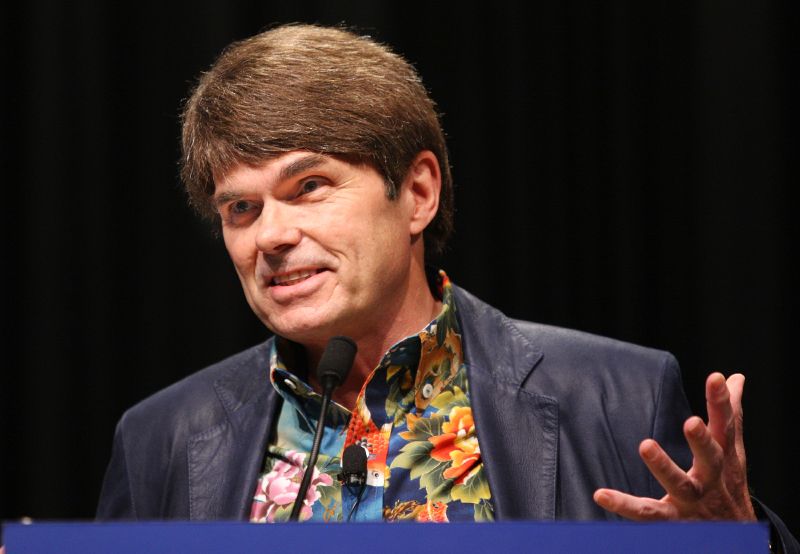A white man, estimated to be around 50 years old, stands on stage speaking to an audience from behind a striking blue podium. Dressed in a black leather coat, he exudes a vibrant presence with a colorful shirt adorned with intricate patterns of flowers and leaves. His blonde hair, resembling the texture of a kiwi fruit, adds a unique touch to his appearance. He is captured mid-speech, smiling warmly, though his gaze isn't directed toward the camera. The backdrop behind him is an abyss of pitch black, providing no additional context or details to the setting. The nature of the event remains uncertain, but it could potentially be a conference or a comic convention, suggested by his enigmatic persona, hinting that he might be an actor or a renowned musician.